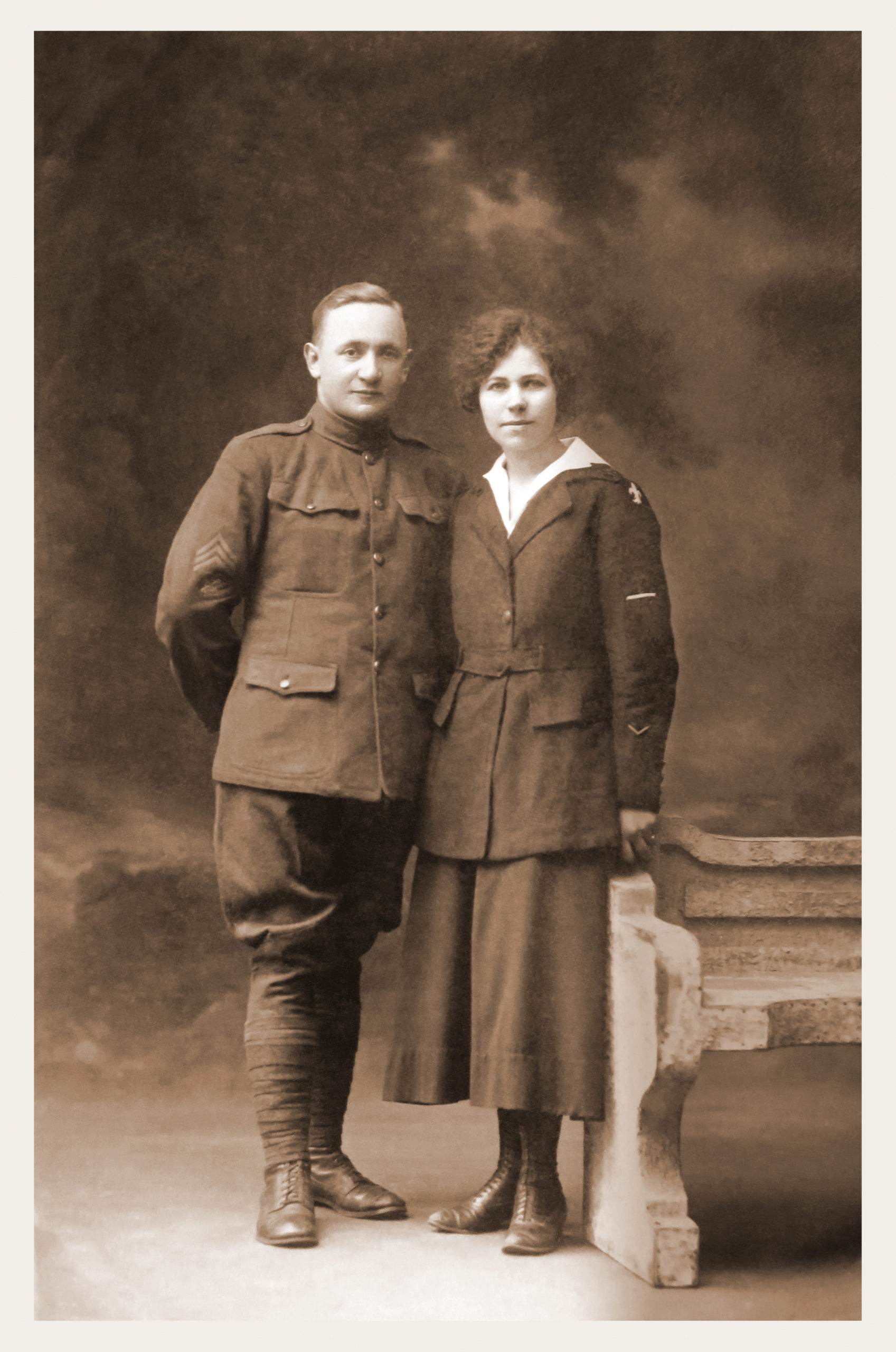This black-and-white portrait photograph, likely taken in the mid-20th century, captures a young couple dressed in formal military attire, standing in a posed and composed manner. The man, positioned on the left, sports a naval uniform with three ranking lines on his right arm. His short, well-groomed hair and long, heavy jacket with baggy trousers and dark shoes give him a distinguished appearance. His stance is formal, with his hands clasped behind his back. The woman, standing on the right, leans gracefully against a stone bench, her hand resting on one of its handrails. She wears a sizeable brown military-style coat over a long skirt, paired with boots, emphasizing her composed demeanor. Her short dark hair frames her face, adding to the formal air of the photograph. The background is blurred and indistinct, featuring what appears to be dark clouds, enhancing the timeless and somber atmosphere of this meticulously staged image.